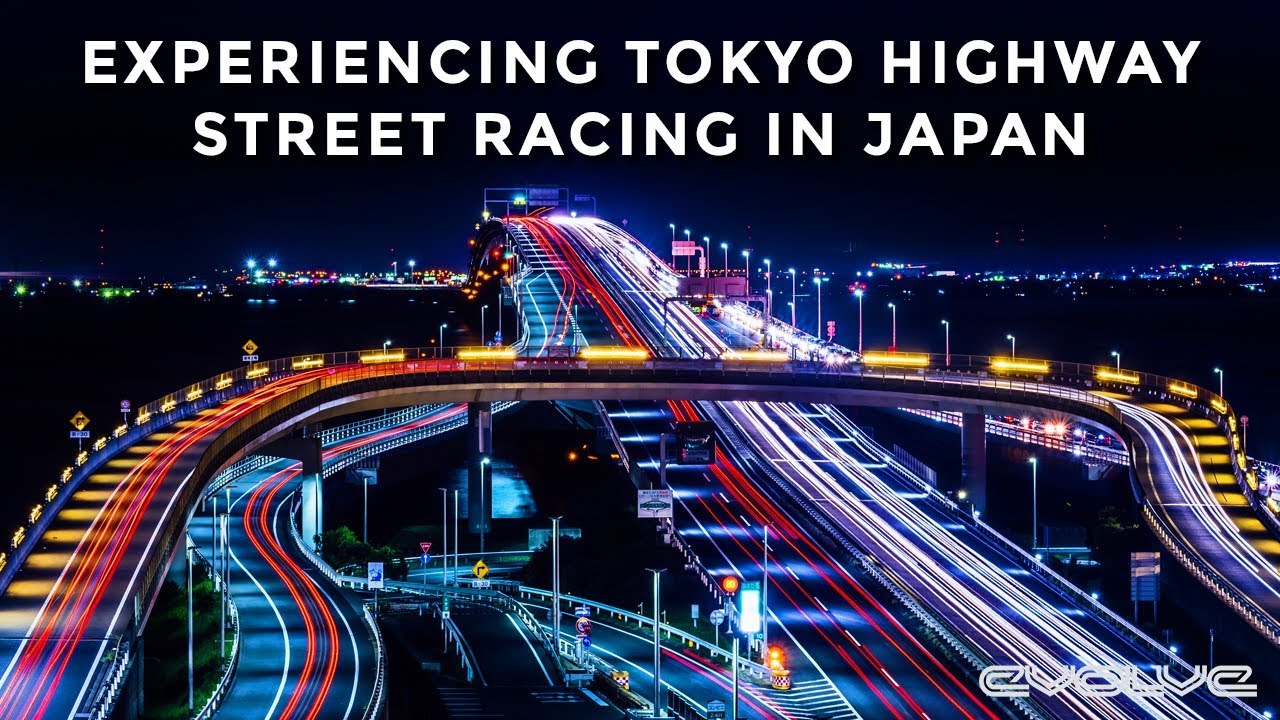The image depicts a vibrant and artistic nighttime scene of Tokyo, Japan. At its top, bold white capital block letters announce, "Experiencing Tokyo Highway Street Racing in Japan." Dominating the foreground is a brightly lit multi-lane highway adorned with neon hues of red, white, orange, yellow, and blue, creating a dynamic streaking effect as if from the motion of racing cars. A large, curving overpass slices through the middle of the scene, casting a shadow over the regular street below, which is illuminated by standard streetlights and adorned with various signs. The background reveals distant city lights that sparkle against a dark blue to black sky, enhancing the sense of depth and urban energy. In the bottom right corner, the word "Evolve" is presented in stylized white block lines, adding a modern and futuristic touch to the composition. The overall effect is a striking, illuminated portrayal of Tokyo's street racing culture set against its iconic cityscape.